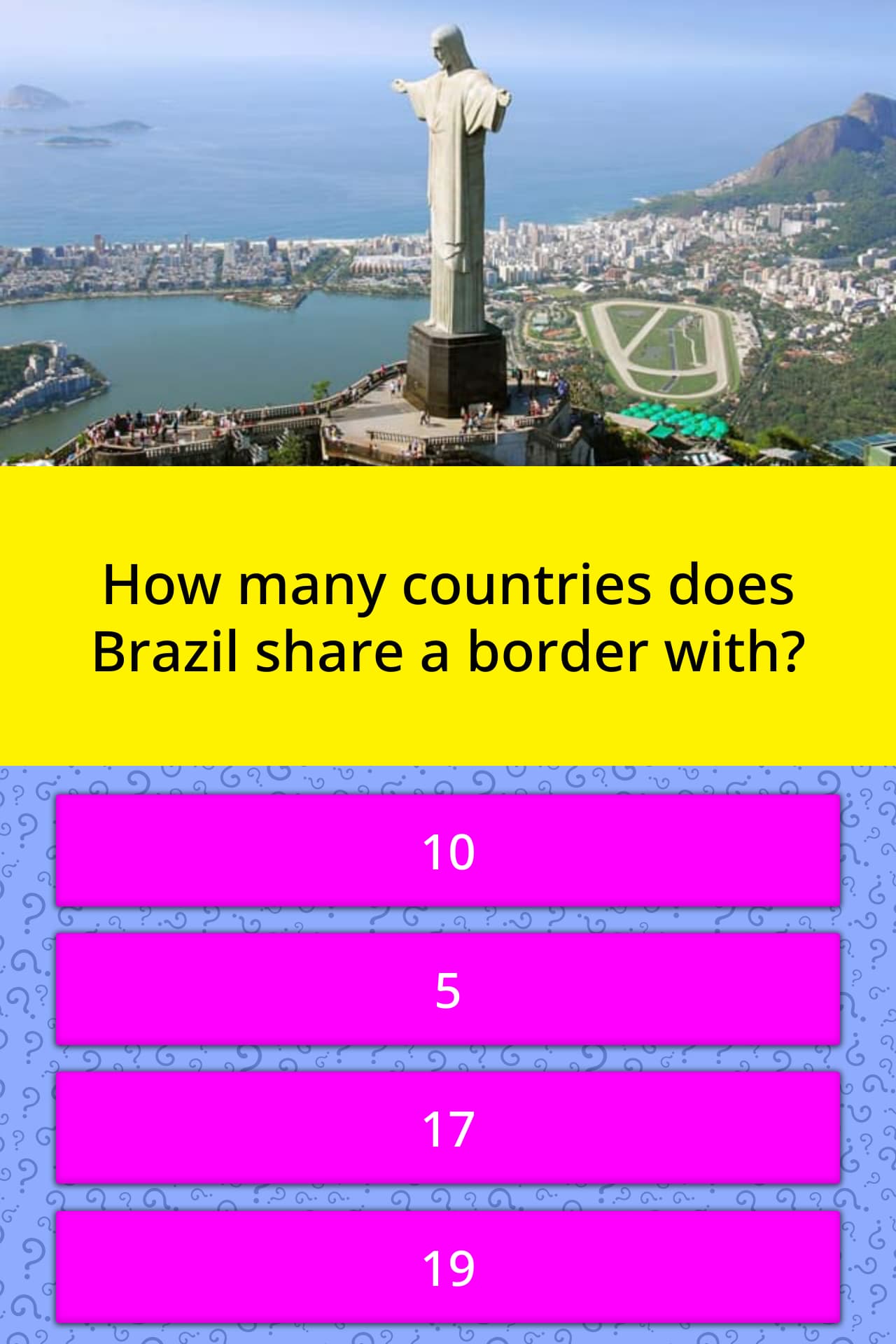Caption: A quiz screenshot featuring a majestic statue of Jesus, dressed in a flowing robe with arms outstretched. The statue, made of white material like marble or cement, is perched atop a hill adjacent to a small walkway and an observation point where people are gathered. Beyond the statue, a vast cityscape with numerous buildings stretches out towards the horizon, with a body of water visible in the distance. A bold yellow band cuts across the center of the image, posing the question, "How many countries does Brazil share a border with?" The possible answers, highlighted in purple, are 10, 5, 17, and 19, inviting users to make a selection to see if they are correct.